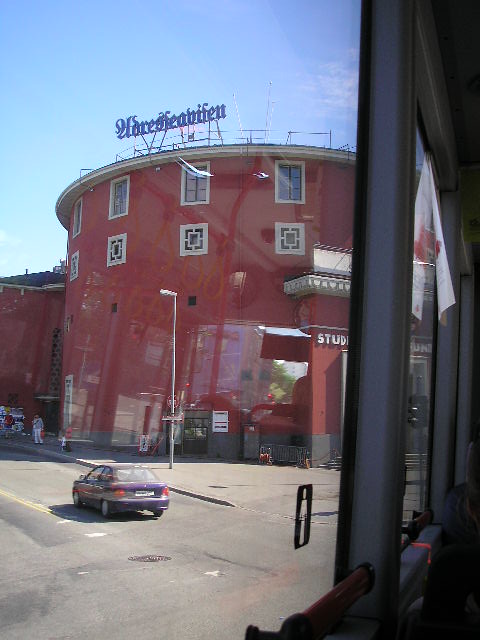The image captures a prominent, cylindrical red building taken from behind a window, likely from a bus, as indicated by the visible reflection. The structure appears to be about four stories tall, with a distinctive roof featuring a rounded top. A sign constructed from pipes and held above the roof reads "Erdendusen," adding a German flair to the scene.

The building's design includes a windowless bottom half, while the upper half is adorned with square windows. These windows consist of alternating white squares and six-paned squares. The sky is bright blue, clearly suggesting it's daytime. In front of the building, a purple car is parked in a lot, along with a visible streetlight and sidewalk. The word "studio" marks the building, and a few people are casually milling about the area.